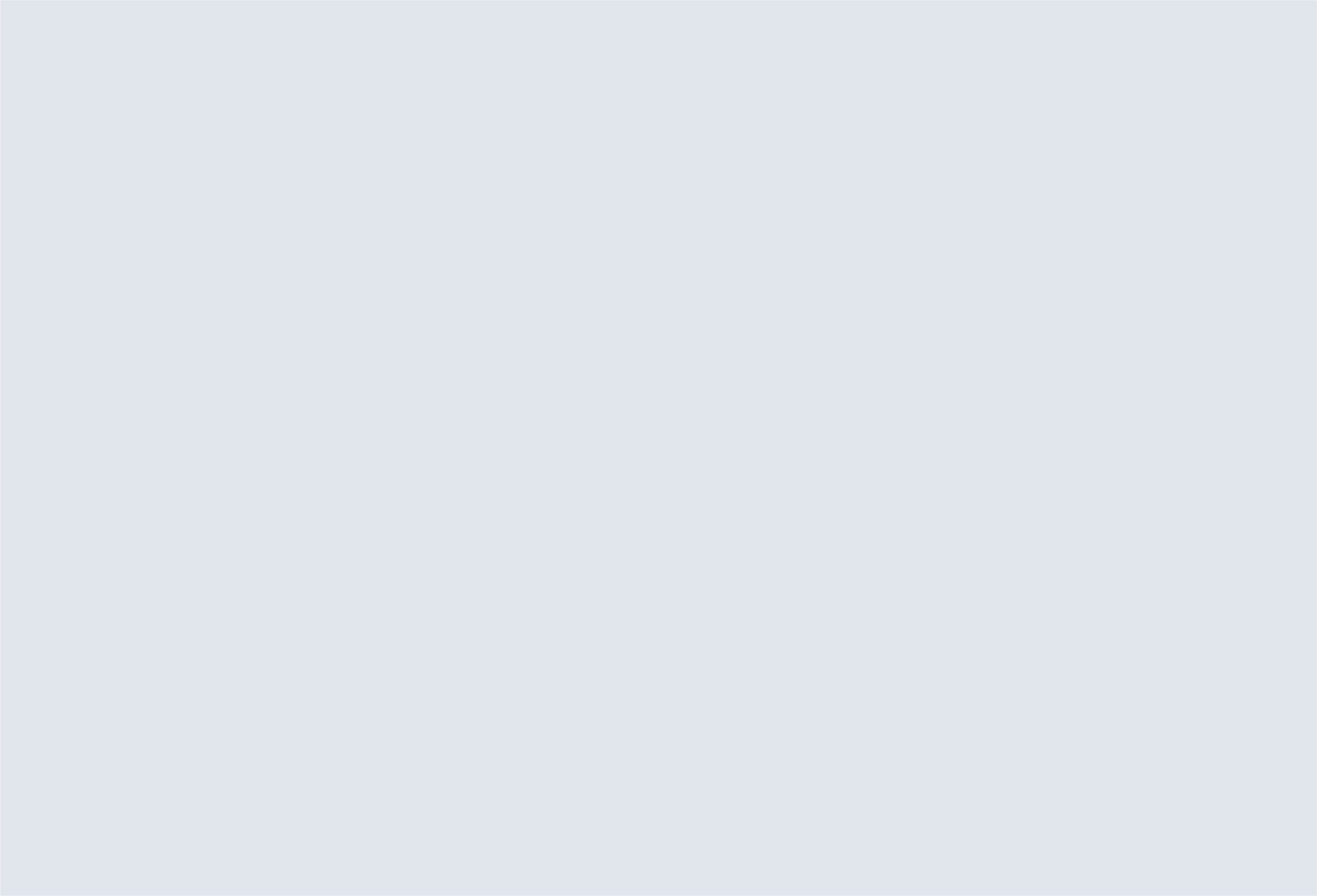A flat, monochromatic gray rectangle fills the entire image. There are no distinguishing features or details within this shape. The gray tone is very light, slightly darker at the top, possibly due to a gradient effect, though it may also be a visual artifact from the monitor contrast. The overall color is subtly darker than the white background of the screen, creating a minimalistic and stark presentation.